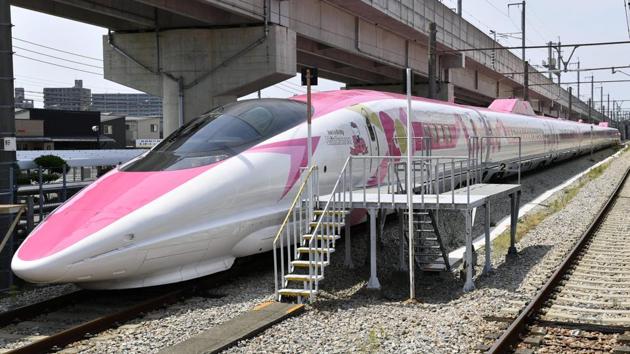In this picture, we see a stationary bullet train characterized by its sleek, aerodynamic design and pointed nose cone. The train features a white body with striking pink accents on the top, along with intricate pink and yellow designs adorning its sides. The front of the train showcases a prominent black windshield. Adjacent to the train, there is a small staircase, white and yellow in color, equipped with poles on either side, presumably leading up to the entrance of the train. The ground surrounding the train is composed of scattered gray pebbles. In the background, a bridge or flyover spans above the train, while to the right, another set of railroad tracks is visible. On the left side, a few distant buildings can be seen, indicating that the scene is set within a city environment.